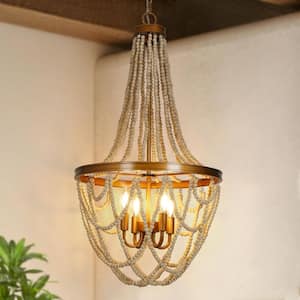The image showcases a chandelier with intricate detailing, primarily featuring gold materials. The chandelier, while modest in size, hangs from the ceiling with a gold bracket that connects it to the ceiling. It features elegant rows of beads cascading into a gold ring, from which further strands of beads hang down, forming graceful loops. Nestled within these loops, five candle flame-shaped light bulbs emit a bright, white light, creating a prominent illumination in the room. The light fixture itself is crafted from brass, gold, or bronze, lending it a rich, warm hue.

The central frame of the chandelier includes several metal rods that provide structural support, branching out to maintain the stability of the beaded loops and bowl-like design. Contrasting with the chandelier's luxurious materials, the surrounding environment exhibits neutral beige walls, a dark brown ceiling that lightens towards a corner, and a hint of green leaves from a plant visible at the bottom left corner of the image. The overall ambiance of the room is enhanced by the chandelier's modern yet classic design, with the white beads and brown or gold frame contributing to its distinctive and elegant aesthetic.